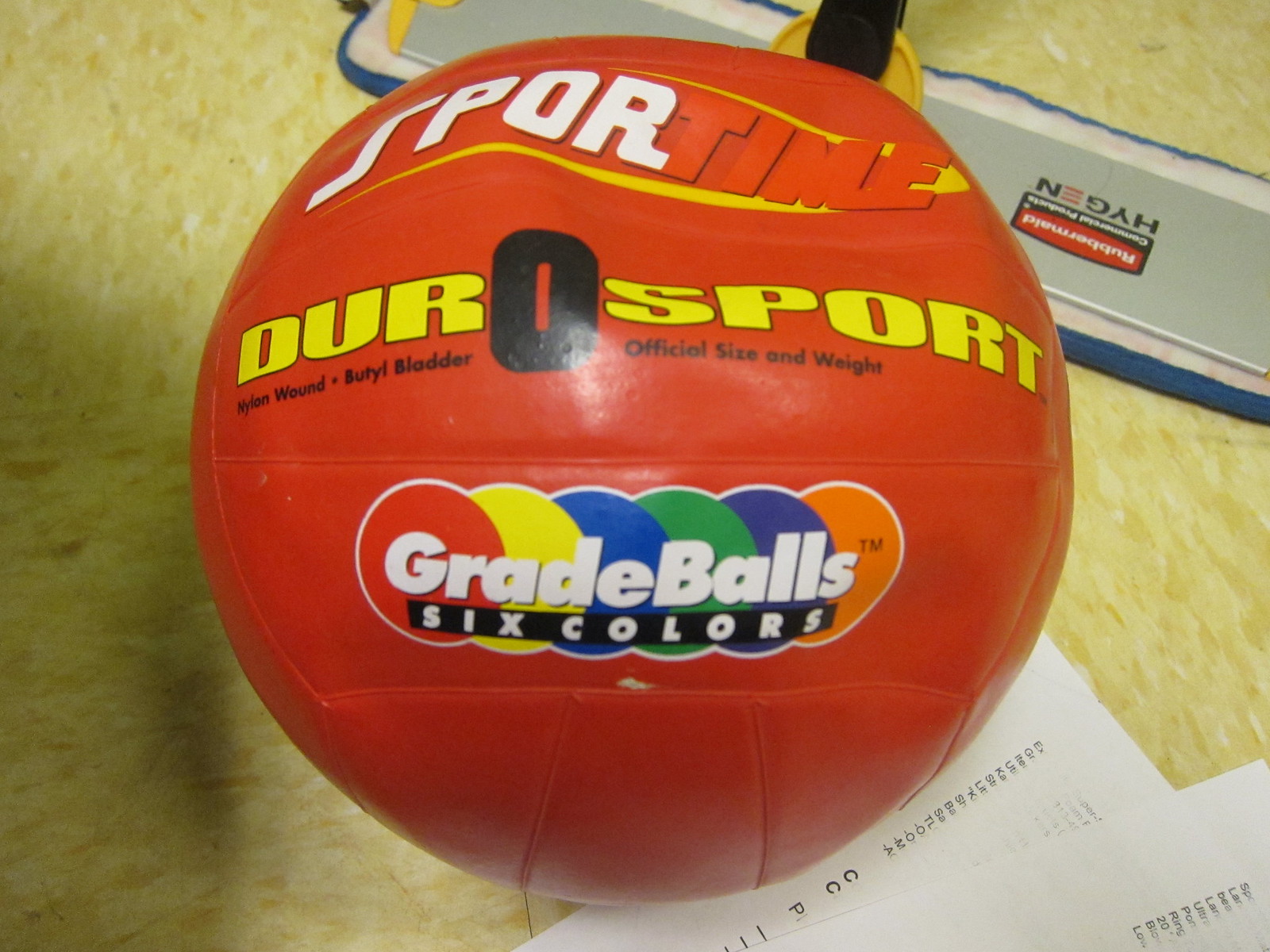This color photo, slightly wider than it is tall, is a close-up of a partially deflated volleyball with a dent in the top right corner, making it appear a little off its official shape. The volleyball is a lighter red, and at the top, it has white and red block letters spelling out "SPORTIME," with "SPOR" in white and "T-I-M-E" in red against a yellow half-oval background. In the center of the ball, it prominently features the brand name "DUROSPORT" in yellow block letters, except for the "O," which is a large black block letter. Below "DUROSPORT," in small, black, printed text, it reads "Nylon Wound Butyl Bladder Official Size and Weight." Further down, in white bubble letters, it says "GRADE BALLS." Behind this text is an array of six balls, each a different color: red, yellow, blue, green, purple, and orange. Beneath them, a black bar contains the text "SIX COLORS" in all capital white letters.